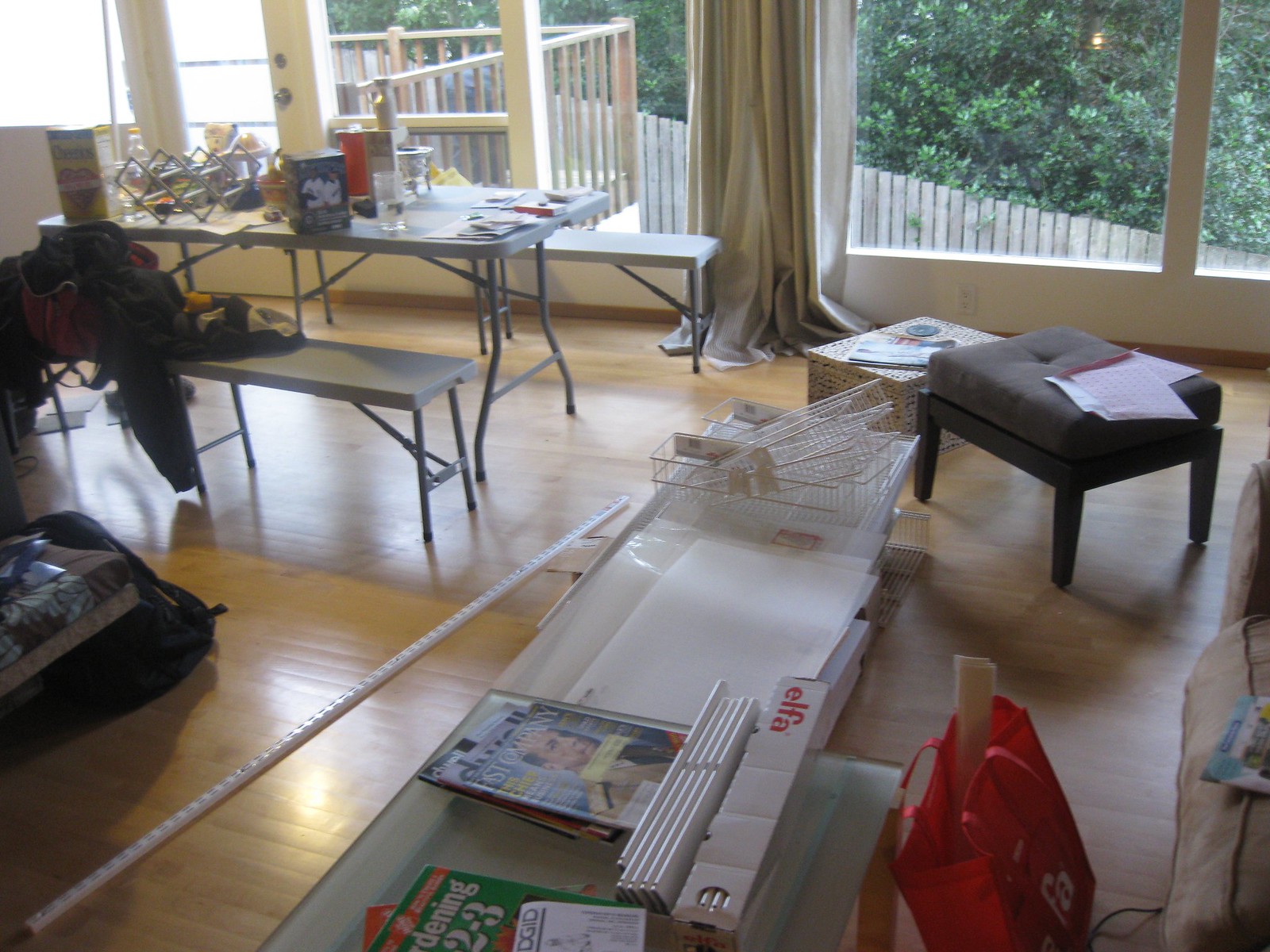Depicting an interior of a residential room, the photograph captures a serene view extending out through a wall of expansive windows. The windows are adorned with open gray curtains, revealing a glimpse of a wooden privacy fence and a lush garden, complete with a patio deck, beyond the glass panes.

Inside, the room features a brown and white hardwood floor. In the foreground, there is a long table cluttered with several items, including a few magazines and plastic containers. A white metal rail lies on the floor in front of this table, adding to the room’s assortment of items.

Centrally positioned across the room is a gray foldable table. It too is laden with various objects, such as cups and boxes. Tucked into a corner sits a brownish footstool, adjacent to which is a cardboard box. Further enhancing the room’s lived-in feel, a red reusable shopping bag hangs behind the foreground table. The overall ambiance is cozy yet functional, indicative of a space used for both relaxation and activity.